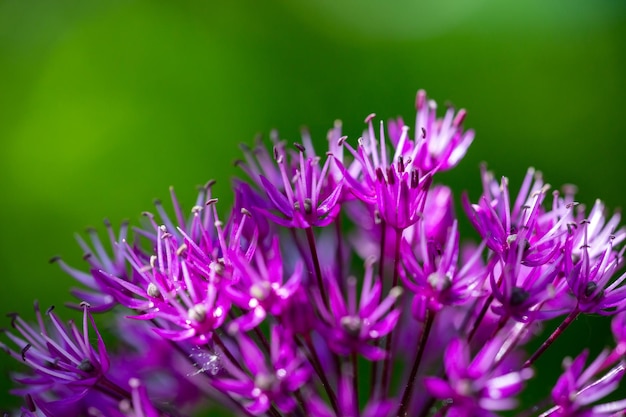This photograph captures a striking display of blooming purple flowers. In the foreground, you see medium purple, spiky flowers with elongated stalks of a dark reddish-purple hue. Each flower features delicate white pistils, topped with deeper purple tips, adding a contrasting intricacy to their appearance. A small spiderweb is visible on one of the bottom flowers, adding a touch of nature's intricacies to the scene. 

The background forms a soft, blurred wash of greenery, ranging from dark forest green to almost a yellowish light green, creating a dreamy, out-of-focus backdrop that enhances the focus on the flowers. The entire scene is delicately highlighted by sunlight, giving the flowers a soft glow. There are multiple flowers in various stages of bloom, showcasing the ongoing cycle of growth and renewal. The dark purple stems and the lilac hearts of the petals make the flowers stand out beautifully against the subtly colored background, making it a captivating and harmonious composition.